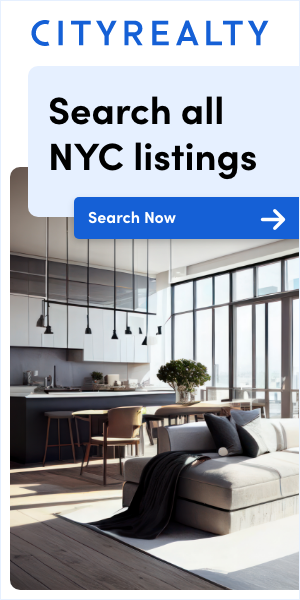The image appears to be a screenshot from the City Realty website or app, with "City Realty" prominently displayed at the top in large blue block-style font against a white background. Below this, there is a light blue text box with bold text that reads "Search All NYC Listings," occupying about a fourth of the image. Beneath this, there is a darker blue button with the text "Search Now" in white font and an arrow pointing to the right. These boxes slightly overlap each other and another image beneath them.

The primary image is a vertical shot of a modern, contemporary apartment. Notable features include hanging lights that resemble torchiere-style fixtures, and a floor-to-ceiling glass door. There is also a kitchen island visible. The apartment has a loft-style design with a couch situated on the right side of the foreground. Behind the couch, there is a rustic country-style table paired with wooden chairs. The flooring is hardwood, enhancing the modern aesthetic of the space.